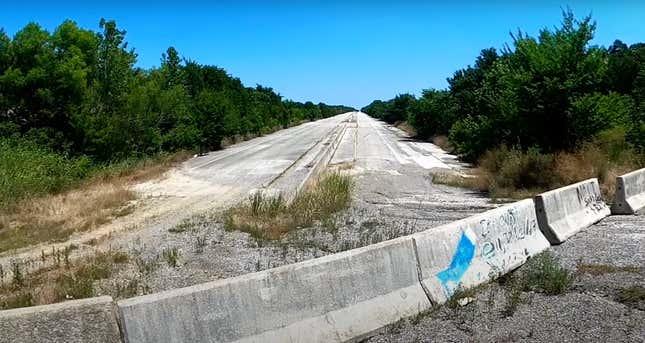This image depicts an abandoned road stretching into the distance under a clear, blue, cloudless sky. Flanked by lush, dark green trees on both sides, the road is lined with patches of green bushes and dry brown grass emerging from cracks in the light gray asphalt, suggesting it has seen better days. In the foreground, a curved set of concrete barriers, marked with indeterminate blue and other colored graffiti, demarcates the entrance to the road. These barriers seem to function as a guard to prevent vehicles from accessing the overgrown and rarely used road. The road itself, composed of weathered gravel and asphalt, meanders slightly from the middle to the bottom right of the photo, enhancing the sense of abandonment and disuse.